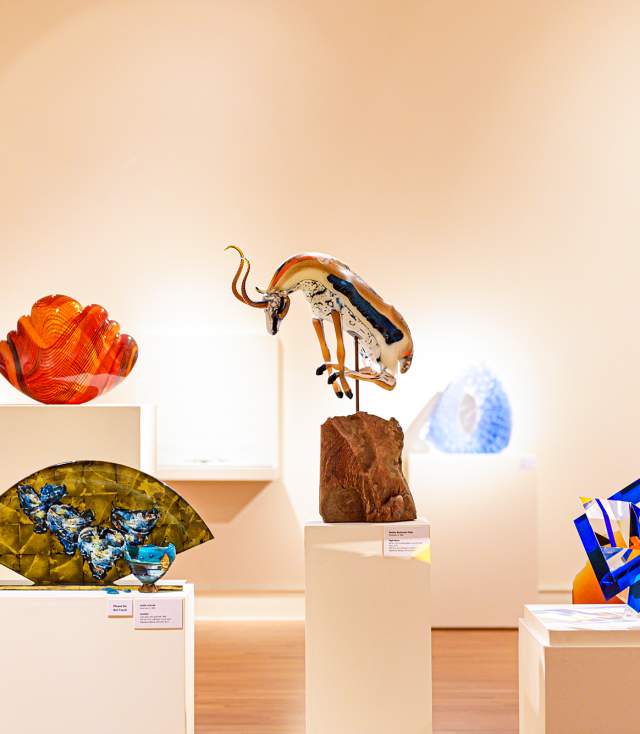The photo showcases a detailed interior of an art museum exhibit with a series of art pieces prominently displayed on pale pink or rosy-colored pillar-like pedestals. The wooden floor adds warmth to the scene, while the background walls are a very light pale pink, tying the exhibit's aesthetic together. To the left, there is an ornate, fan-like structure, adorned in golden and blue hues, which could be a napkin holder with floral elements. Beside it, an orange, glossy object, possibly a gemstone, stands out.

In the center of the image, a striking sculpture depicts a leaping stag or deer, characterized by a body painted in brown and white, with a black patch on its side. This dynamic figure appears to be vaulting over a rough, brown rock-like base, giving a sense of movement to the display.

On the right side of the exhibit, a large, sky-blue, globular shape is noticeable in the background. Further to the right, in the bottom foreground, there is a geometric structure made of dark blue glass, which contrasts with another blue and white glass object visible towards the back right of the image. Despite the small placards that provide information about each artwork, their texts are too small to be legible in the photograph. Overall, the exhibit combines the elements of color, form, and texture to create an engaging and visually harmonious display.